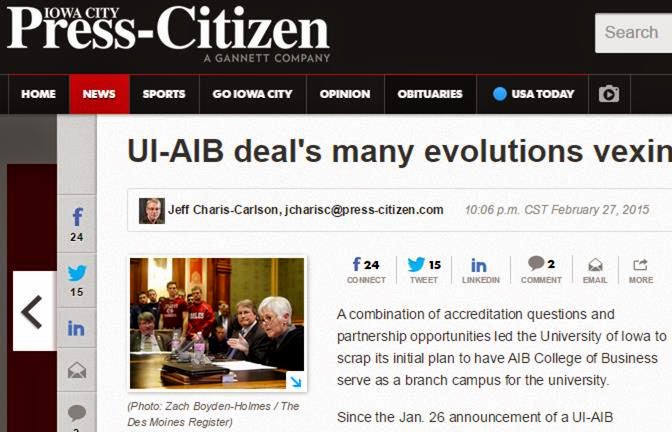The image is a partial screenshot from the upper left quarter of a website belonging to the Iowa City Press-Citizen. At the very top, there is a dark banner featuring the text "Iowa City" in white. Prominently displayed beneath it in larger white text is the title "Press-Citizen," followed by the tagline "A Gannett Company" in smaller white letters.

To the right of the banner, there's a visible search box. Below this banner lies a navigation bar consisting of clickable tabs for different sections: Home, News, Sports, Go Iowa City, Opinion, Obituary, and USA Today. The News tab is distinctly highlighted in red, indicating it is the selected section, while the others remain against a black background.

The main article’s headline is partially visible and reads, "UA-AIB deals many evolutions vexing [cut off]." Beneath the truncated headline, the article includes a photograph depicting a group of white individuals sitting at a table engaged in conversation.